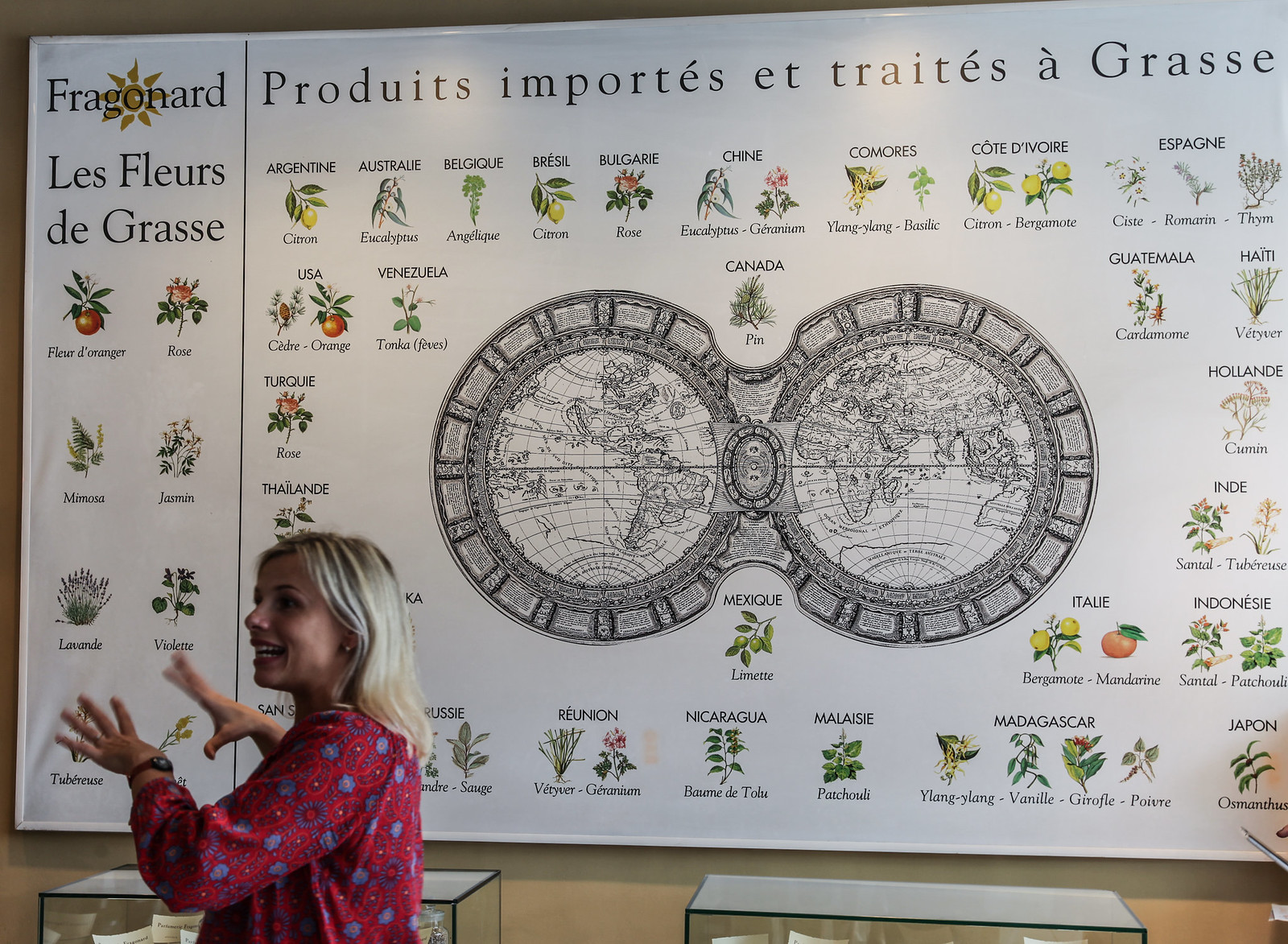This image captures a woman standing in the bottom left corner, her blonde hair falling just past her shoulders. She's wearing a red blouse adorned with purplish-blue circular patterns. Her arms are raised halfway, gesturing animatedly, suggesting she might be explaining something to an unseen audience. Behind her stretches a large, detailed poster measuring approximately 15 feet wide and 6 feet high, featuring various types of plants, herbs, and fruits accompanied by their names in French. Dominating the center of the poster is a vintage black-and-white world map. The poster includes text such as "Fragonard Produits Imports et Traits Gras" and "Les fleurs de gras." The backdrop is a beige wall with intermittently visible display cases below the poster, their tops outlined in black. The overall scene gives the impression of being set in a classroom or museum, emphasizing the educational nature of the setting.